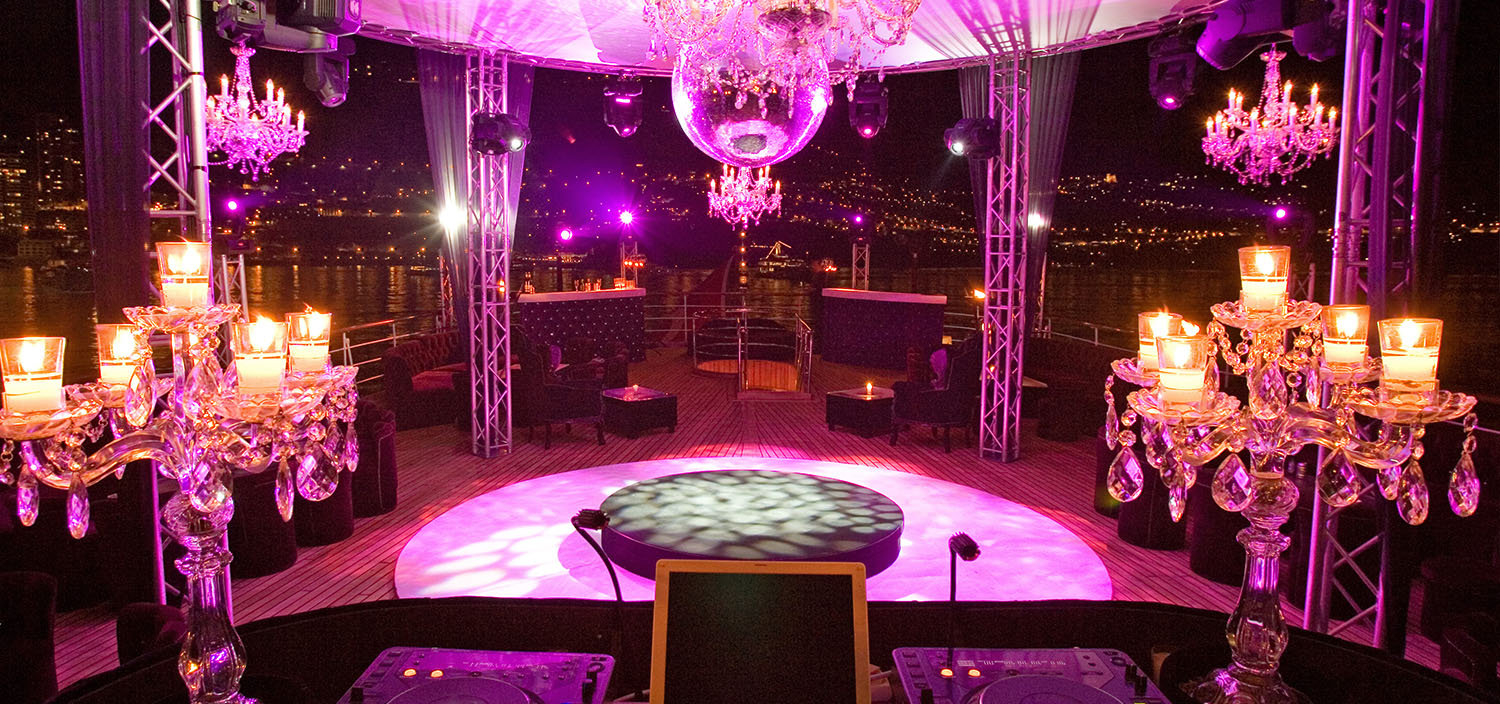The image portrays a luxurious, semi-outdoor setting illuminated by elegant lighting. The scene is dominated by a central area with a circular cushion laid out on a hardwood floor, accompanied by a carpet. This area is bathed in a violet-purplish light emanating from a see-through orb hanging in the top center. Floor-to-ceiling windows frame the area, revealing a sprawling city skyline and a large body of water in the far distance, giving the setting an appearance that could be akin to the deck of a ship or a waterfront location.

The main focal point is a central stage-like structure, featuring a monitor and turntables on either side at the bottom center, flanked by ornate, glass candlesticks. Flanking the area on the left and right are intricate crystal chandeliers, with a larger chandelier also suspended in the top center, casting a mesmerizing pink and purple glow throughout the space. Additional warm yellow light is provided by numerous lit candles in crystal candelabras, each holding five candles, positioned on side tables. The overall ambiance is one of opulent elegance, enhanced by the interplay of warm candlelight and cool magenta illumination, creating a captivating and sophisticated atmosphere.